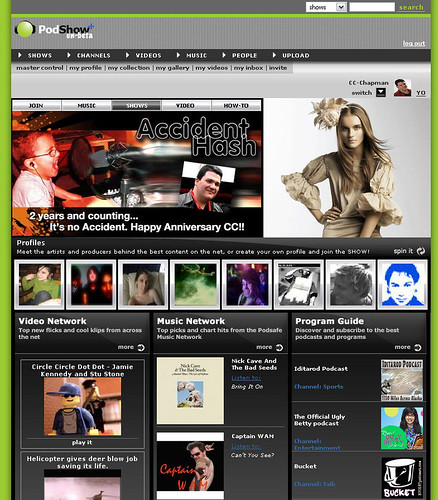This is a screenshot taken from someone's computer displaying a web page. At the top of the screen, there's a navigation bar with a green circle logo labeled "Pod Show." It includes menu options such as "Shows," "Channels," "Videos," "Music," "People," and an "Upload" button. The green circle at the top features a thin line extending above it which culminates in a word search field in the same green color.

On the left and right sides of the screen, vertical green lines are visible—the line on the left is slightly thicker compared to the one on the right. Below the navigation bar, there's a section titled "Accident Hash," which is identified as a show with a tagline reading "Two Years and Counting. It's No Accident. Happy Anniversary CC."

Beneath this title, there are a few images. The first image appears to depict a young child wearing ear pods or wired earphones, enthusiastically screaming into a microphone. Next to this image is a picture of an adult man, possibly indicating who the child has grown into. Additionally, there is an image of a woman adorned in a frilly dress with a fuzzy accessory on her head.